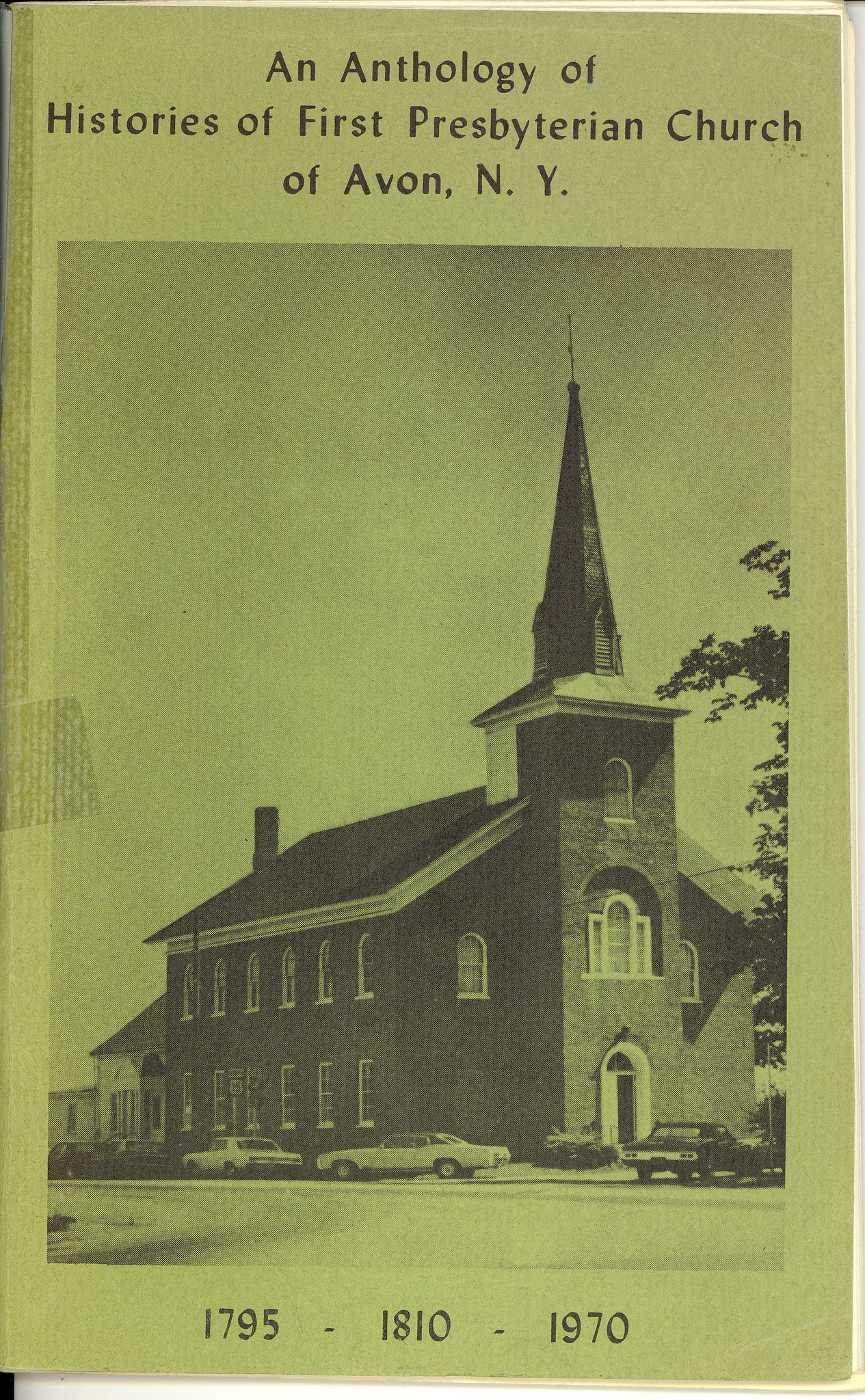The front page of this book, titled "An Anthology of Histories of First Presbyterian Church of Avon, NY," is prominently displayed at the top. The cover is a dark, faded green color, and it features a black-and-white image of a large, two-story brick church with a towering steeple topped by a cross. The front door of the church is open, and several cars, which appear to be from the 1970s, are parked in front of and beside the church. Notably, the car directly in front of the church is black, while two white cars are parked to the side. Visible trees frame the scene, adding to the historical atmosphere. The lower part of the cover lists the years 1795, 1810, and 1970, highlighting significant dates in the church's history. There is a number 15 visible on the side of the church, adding another layer of detail to the image.